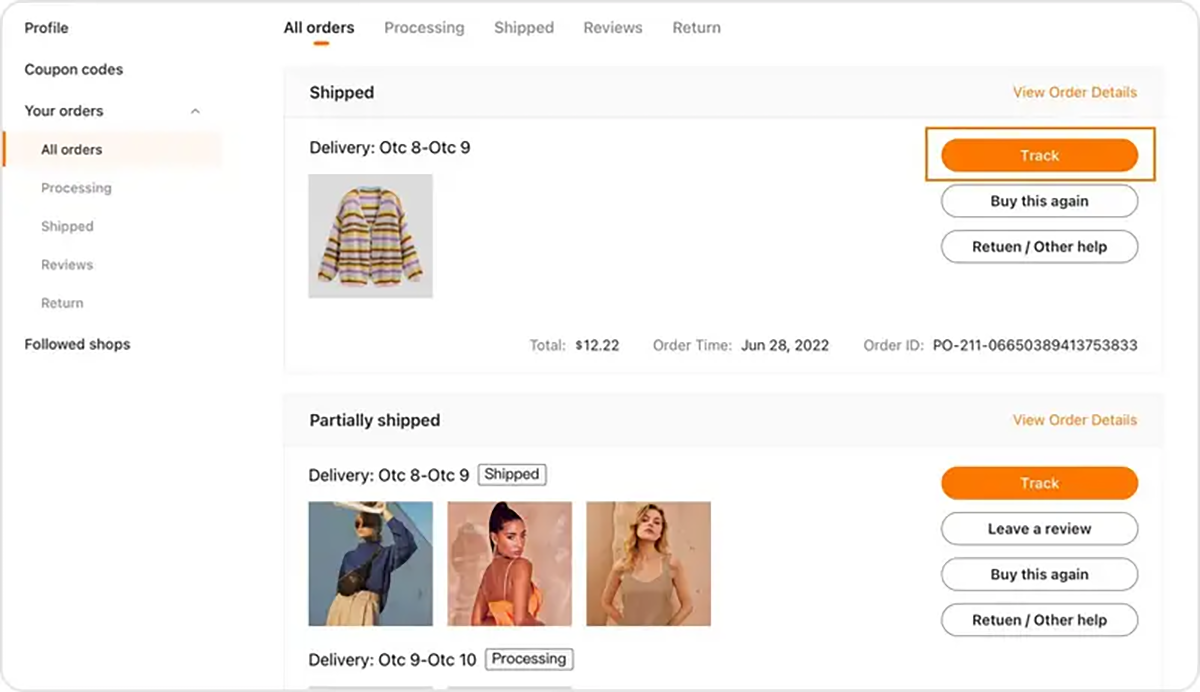Screenshot of an Anonymous Order Page: Detailed Description

This image is a screenshot of an order page from an unspecified website, as there is no distinguishable branding present. 

On the top left corner, the navigation panel displays four tabs arranged vertically in the following order: Profile, Coupon Codes, Your Orders, and Followed Shops. The tabs labeled 'Profile' and 'Coupon Codes' are collapsed, while the 'Your Orders' tab is expanded, indicated by a small gray triangle pointing upwards. Beneath the 'Your Orders' section, there are subcategories listed in smaller text: All Orders, Processing, Shipped, Reviews, and Returns. The 'All Orders' subcategory is highlighted in orange with an adjacent orange bar, indicating the current active view.

The main content area to the right of the navigation panel provides a detailed breakdown of the user's orders within the 'All Orders' subcategory. The orders are displayed in individual rectangles. The first order lists a sweater, identified by a thumbnail image on the left side of the rectangle. Above the thumbnail, the order status is displayed as "Shipped," with the delivery date mentioned just below the status.

On the far right of this order's rectangle, options such as 'View Order Details,' 'Track,' 'Buy This Again,' and 'Return' are available. Additional order details, including the total amount, order time, and order ID, are shown in smaller black text beneath these options.

Below this first order, another section displays an additional order comprising three different items, following the same layout and format. Each item is similarly detailed with corresponding thumbnail images, statuses, and action buttons for further management of the orders.